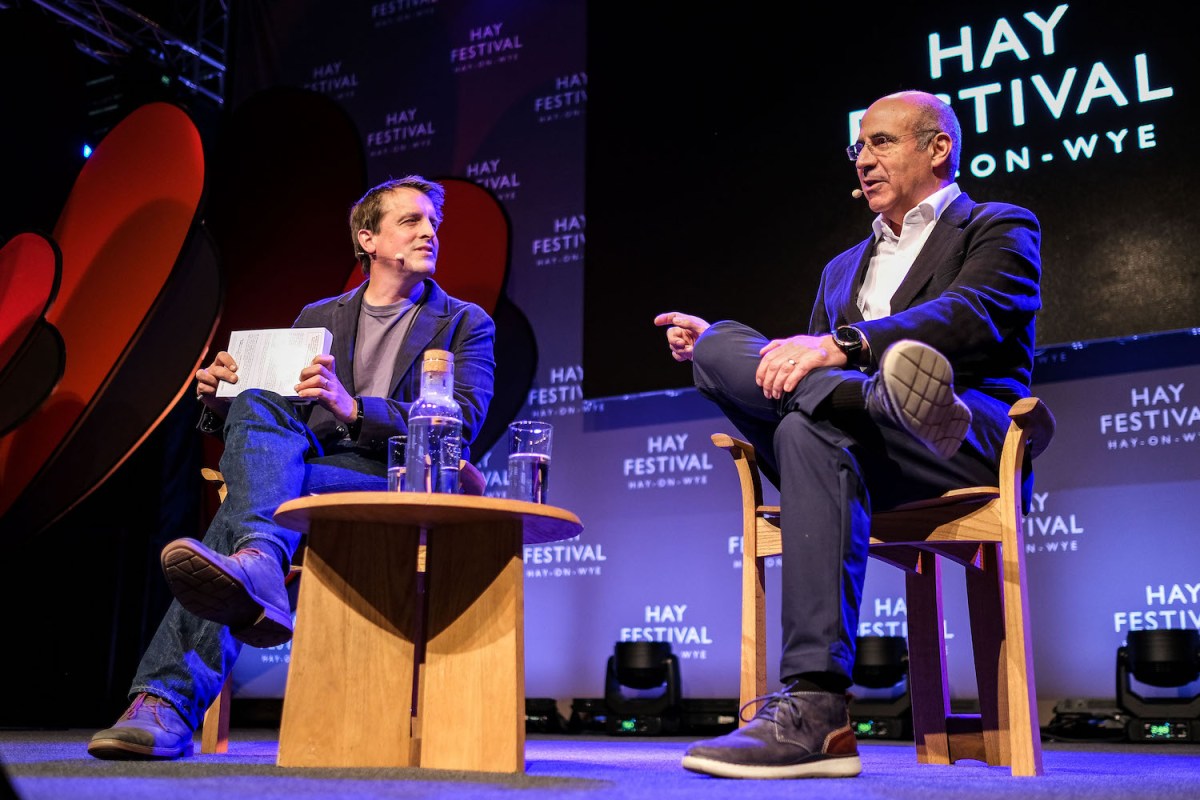The image captures two Caucasian men on stage at the Hay Festival in Hay-on-Wye. The backdrop and a large monitor prominently display the festival’s logo. The scene has a cozy atmosphere with a spotlight illuminating the stage. Both men are seated on wooden chairs with a small round wooden table with a carafe and two glasses of water between them. The man on the left, wearing a gray shirt, gray coat, and blue jeans, sits attentively with his leg crossed and holding papers, seemingly prepared for a discussion. He listens intently to the older man on the right, who sports a white button-up shirt, gray jacket, gray pants, and tennis shoes. The older man, balding and wearing glasses, appears to be speaking. Both men are equipped with headsets, suggesting a live discussion, interview, or podcast recording. The stage is subtly colored in maroon, blue, gray, white, yellow, and black.